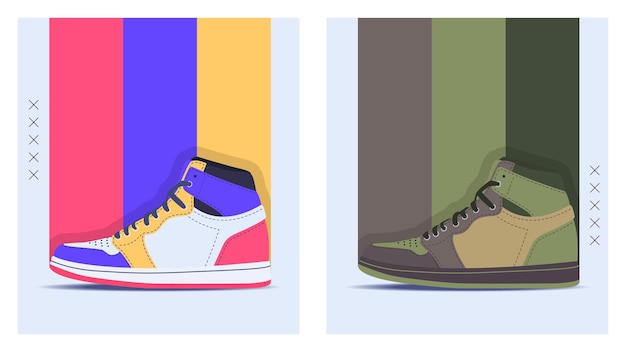The image features two side-by-side sneakers set against a light blue background, each bordered by five X's along the side. The left sneaker exhibits a vibrant design with wide straps of red, blue, and yellow stretching across its entire width. The shoe itself incorporates these colors along with striking white panels. Key details include a blue front panel, stitched yellow segments with white, predominantly white upper sections, dark shoelaces, and a fine red trim at the bottom. On the right, the sneaker displays a blend of three different shades of green, complemented by tan elements, creating a camouflage-like effect. This shoe features dark green, light green, and dark gray panels, light brown sections, and a black trim on the bottom. Both shoes appear to be rendered through a painting or computer animation, presenting a stylized, sporty look.